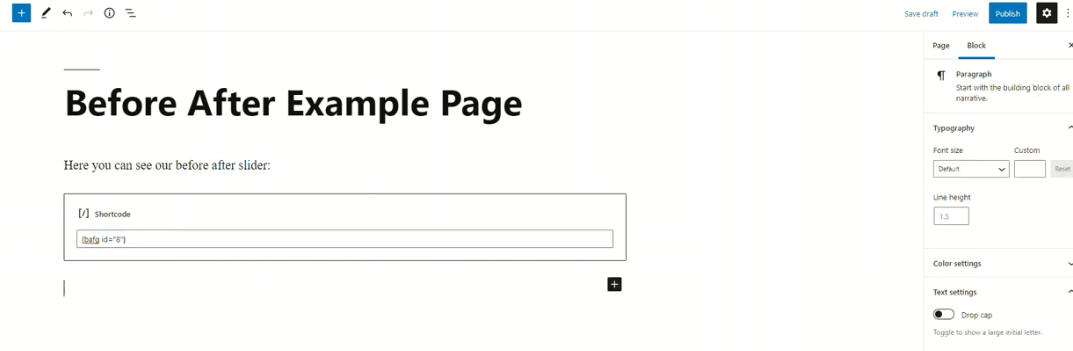A small, blurry screen capture showcases a minimalistic interface, likely from an application or website. At the top, a series of icons are displayed, the specifics of which are indiscernible due to the image's low resolution. The screen is labeled with the words "Before," "After," and "Example Page," hinting at a comparison feature. The phrase "you can see one" is partially visible, followed by an illegible term ending with "slider," implying there might be an interactive element allowing users to toggle between different states, such as before and after views. The background is predominantly white. On the right side of the screen, additional buttons are seen, possibly including a settings option. The overall page appears sparse and plain, with insufficient visible details to determine its exact purpose or the software it belongs to.